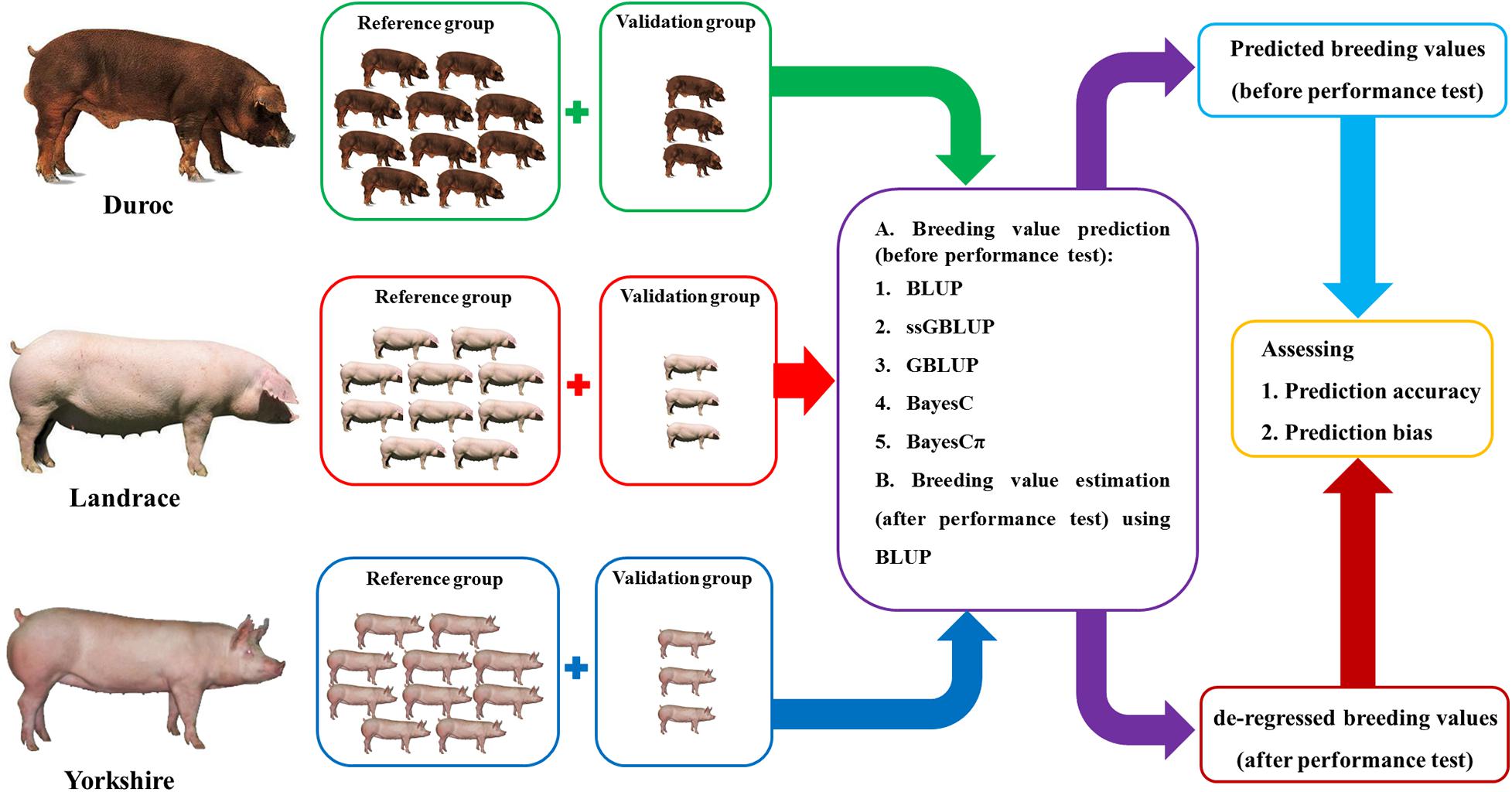The image is a detailed infographic illustrating the breeding value prediction process for three different pig breeds: Duroc, Landrace, and Yorkshire. Each breed is represented with images and divided into reference groups and validation groups. The reference groups show a larger number of pigs, while the validation groups contain three pigs per box. The flowchart includes arrows and rounded squares with text explaining the steps in the process. The first step involves breeding value prediction before the performance test, featuring various prediction methods like BLUP, GBLUP, Bayes C, and Bayes C, Pi. The next step is breeding value estimation after the performance test using BLUP. Following this, the infographic presents predicted breeding values before the performance test, assessment of prediction accuracy, and prediction bias. The final component is the de-regressed breeding values after the performance test. This complex diagram effectively communicates the stages involved in evaluating and predicting breeding values in pig production, focusing on Duroc, Landrace, and Yorkshire breeds.